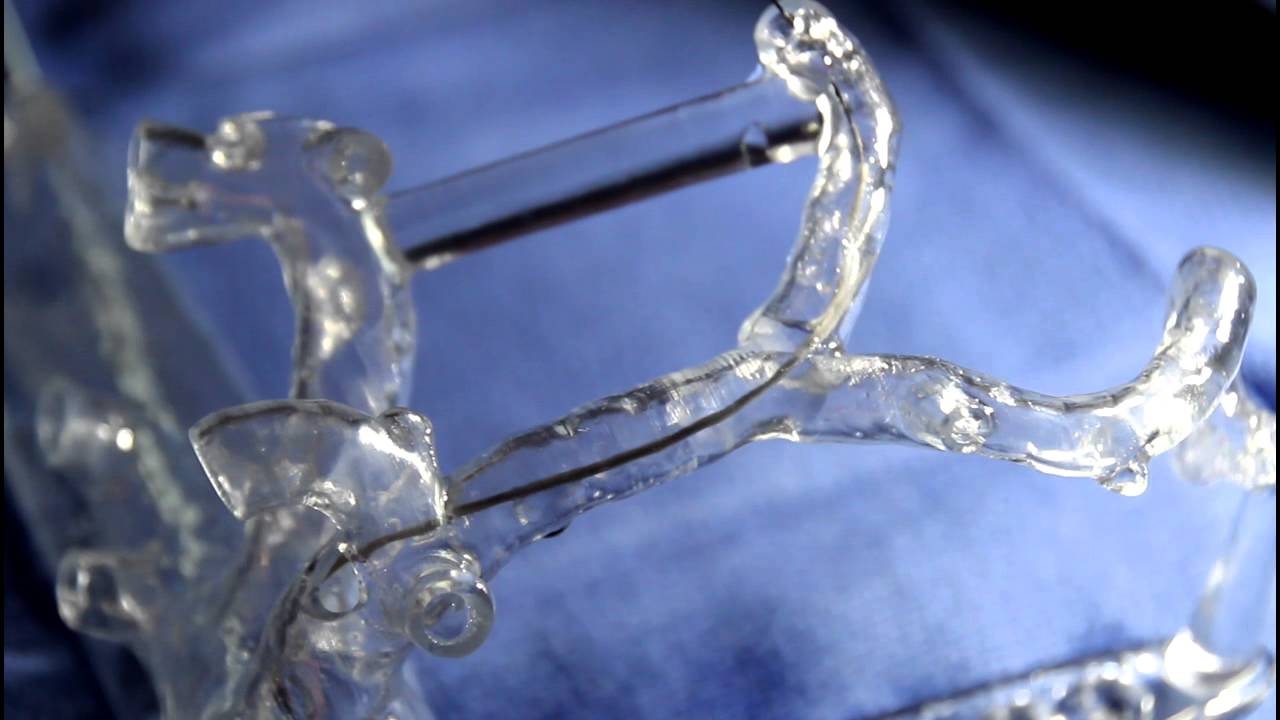This close-up, zoomed-in color photograph showcases a complex glass sculpture against a dark blue and partially black background. The sculptural piece features a network of curved, clear tubes, likely made of glass given the thickness of the material and absence of moisture, hinting it might be an ice-like but dry sculpture. The glass appears intricate, with parts resembling a long, thin tube that splits and curves on the right side, and a longer piece in the background suggesting the head and neck of a dragon or lion. Some sections of the sculpture show small holes, potentially functional or a detail distorted by the photograph’s perspective. Highlighting the right part of the image is a bright light reflecting off the glass, adding to the sculpture's ethereal quality. The background includes a blue cloth with periwinkle hues, though it seems slightly out of focus, with the top right blurring into black. The overall effect is a mesmerizing and abstract interplay of light, glass, and shadow, although the exact nature and form of the sculpture remain ambiguous.